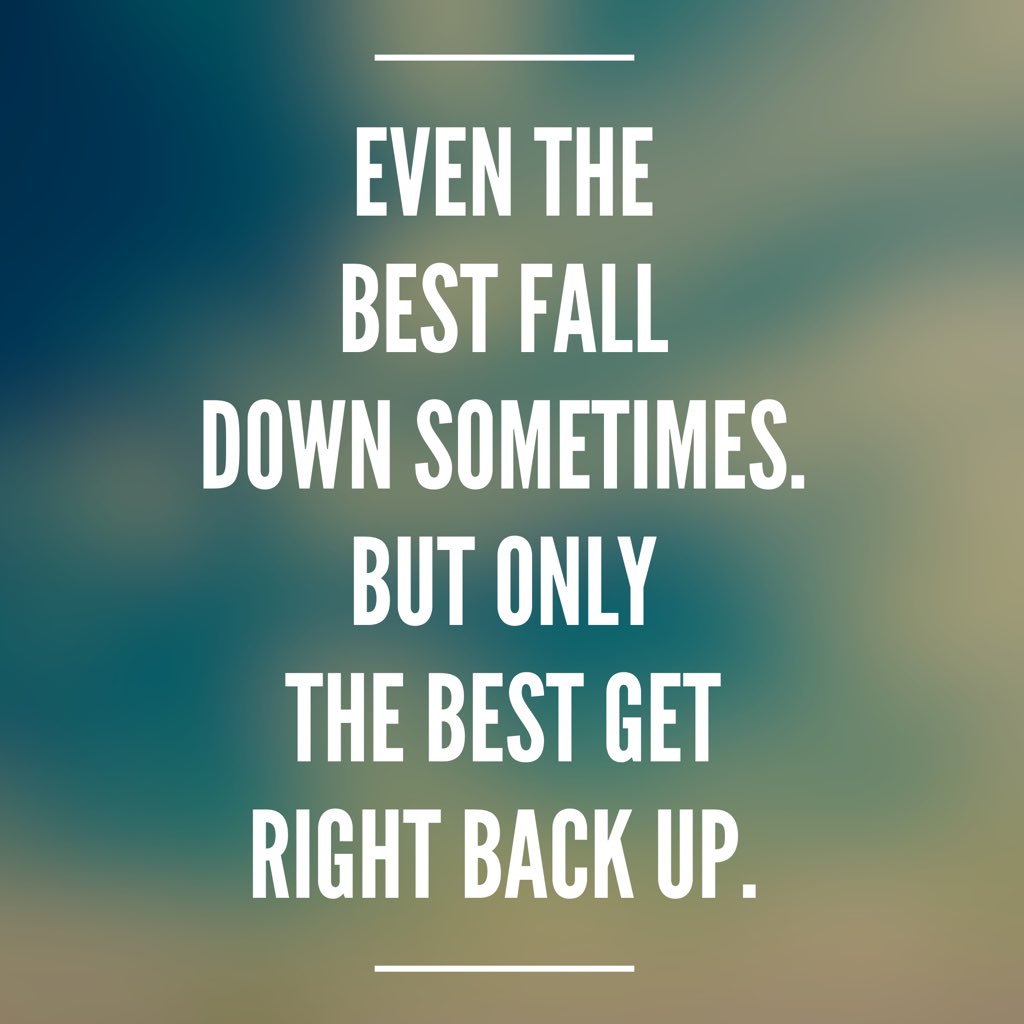The image is a vertical rectangle featuring a fuzzy, blurred background that appears to be a light blue sky with white clouds mashed together, particularly noticeable on the right-hand side. At the top and bottom of the image, there are horizontal dashed white lines framing six centered lines of text. The text, written in all capitalized white block letters, reads: 

"Even the
 Best fall
 Down sometimes.
 But only
 The best get
 Right back up."

The lines are evenly spaced and center justified, creating a visually balanced composition with ample empty space reinforcing the motivational nature of the message. The background colors include shades of blue, white, and hints of green and tan, further enhancing the inspirational tone of the quote.